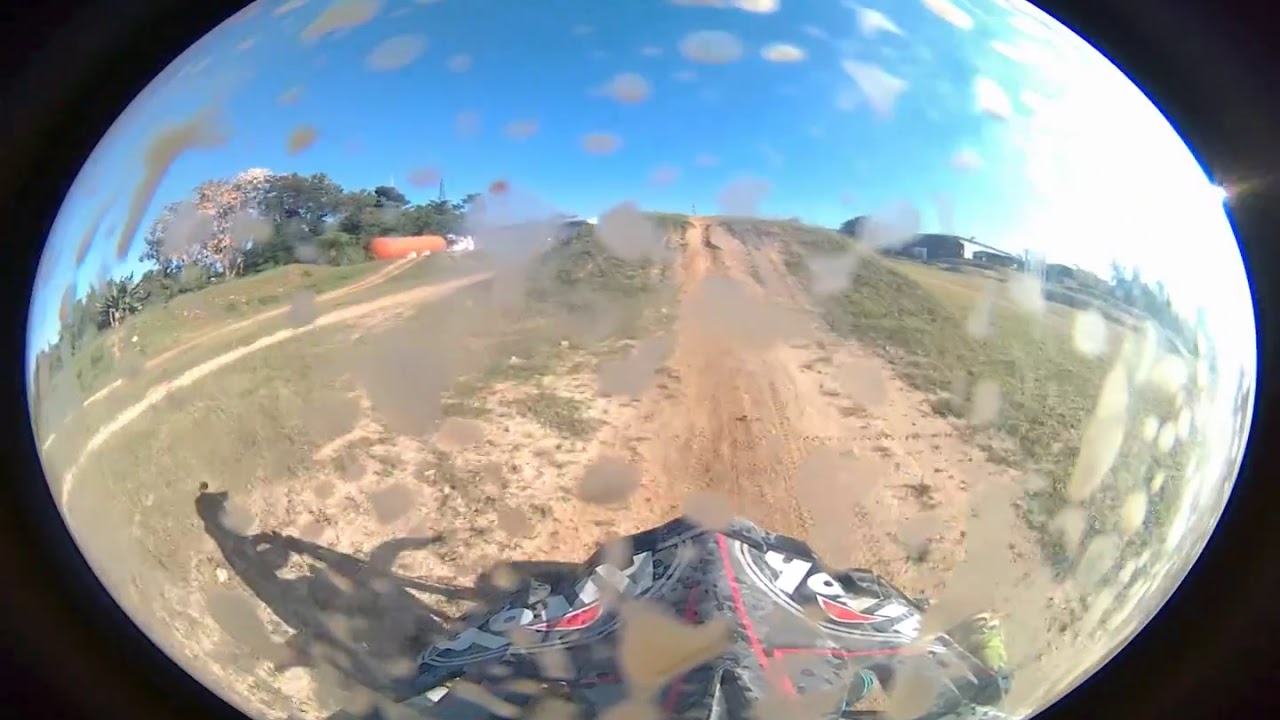The image appears to be captured using a GoPro or similar action camera mounted on a motorcycle helmet, producing a circular picture with noticeable fishbowl distortion. The lens is partially splattered with mud, affecting the clarity. At the center, a brownish dirt road stretches ahead, framed by lush green hills and fields on either side. The upper portion features a striking blue sky, interspersed with a few white clouds, contrasting with a sun-blown segment in the upper right quadrant. A grove of green trees is visible in the upper left quadrant. The composition includes the black, white, and red front of the motorcycle prominently in the lower part of the image, alongside the shadow of the bike and rider extending towards the left lower quadrant. There appears to be an orange truck with a barrel in the background. The entire scene is dynamic and vividly captures the essence of an adventurous ride through a picturesque landscape.